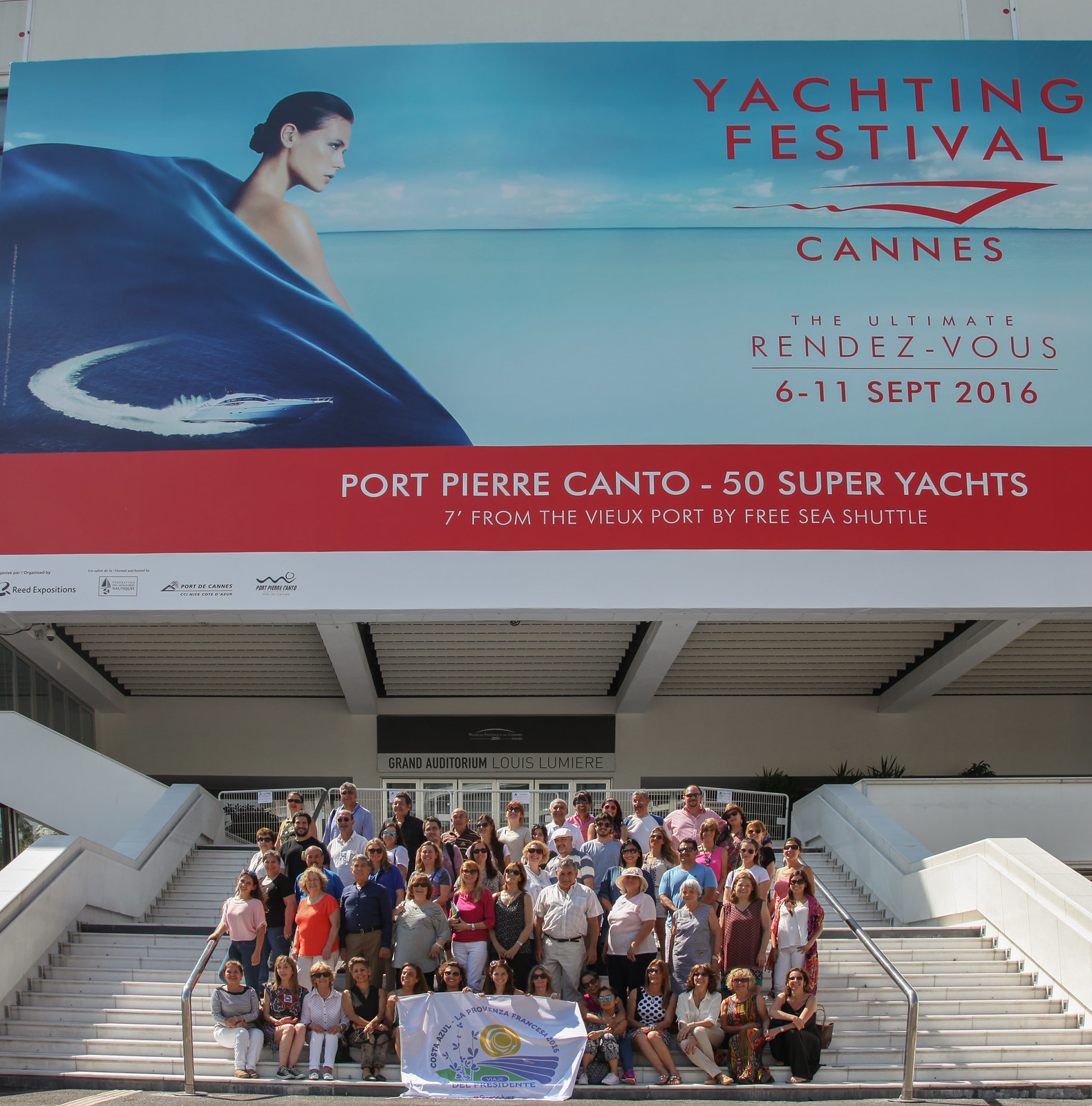A large group of approximately 50 to 60 people are captured in a photo taken on a grand staircase. The group comprises a diverse mix of men and women, spanning a wide range of ages. They are arranged in about five or six rows, with the first row seated on the steps and the others standing behind them. Prominently, the women sitting in the front row hold a large white banner adorned with a sun, a body of water, and grass. This banner adds a focal point to the composition.

Behind the group, a building's wall features a large advertisement for the "Yachting Festival Cannes," which took place from September 6th to 11th, 2016. The advertisement showcases an idyllic beach scene with a woman draped in a blue sheet that transitions into water, complete with a boat sailing on it. Bold red text on the ad reads, "Yachting Festival Cannes, the ultimate rendezvous," and below that, a red bar states, "Port Pierre Canto, 50 super yachts, 7 ft from the Vieux Port by Free Sea Shuttle." This visually striking ad frames the group and adds context to the event they are attending.